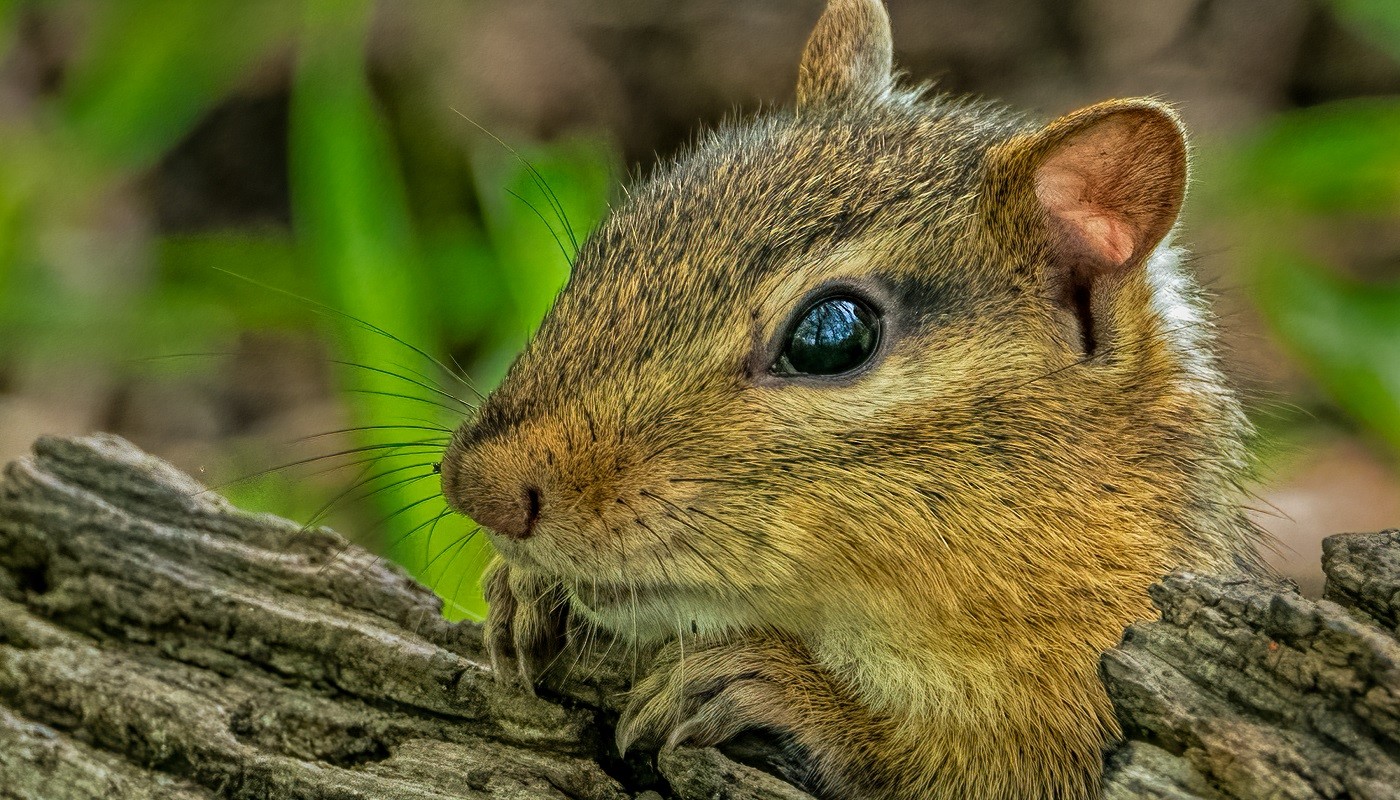This photograph captures a close-up of a small woodland creature, likely a squirrel or chipmunk, perched on what seems to be a log or perhaps a piece of fallen wood. The cute critter's face dominates the image, with its big, dark eyes looking intently towards the left. Its tiny, round ears have a pink inner lining, clearly visible on the ear closest to the camera. The fur is a blend of brown, gray, and orangish hues, transitioning to a lighter, almost white shade under its mouth. The creature's nose is twitchy, adorned with long black whiskers sprouting from both sides, though more sparsely on the cheeks.

It grips the log with its front paws, which are positioned in front of its face, showing off sharp nails at the ends of its fingers. The creature's mouth is slightly open, adding to its inquisitive expression. Behind it, the background is a blurry mix of green and brown, suggesting a woodland area with foliage.